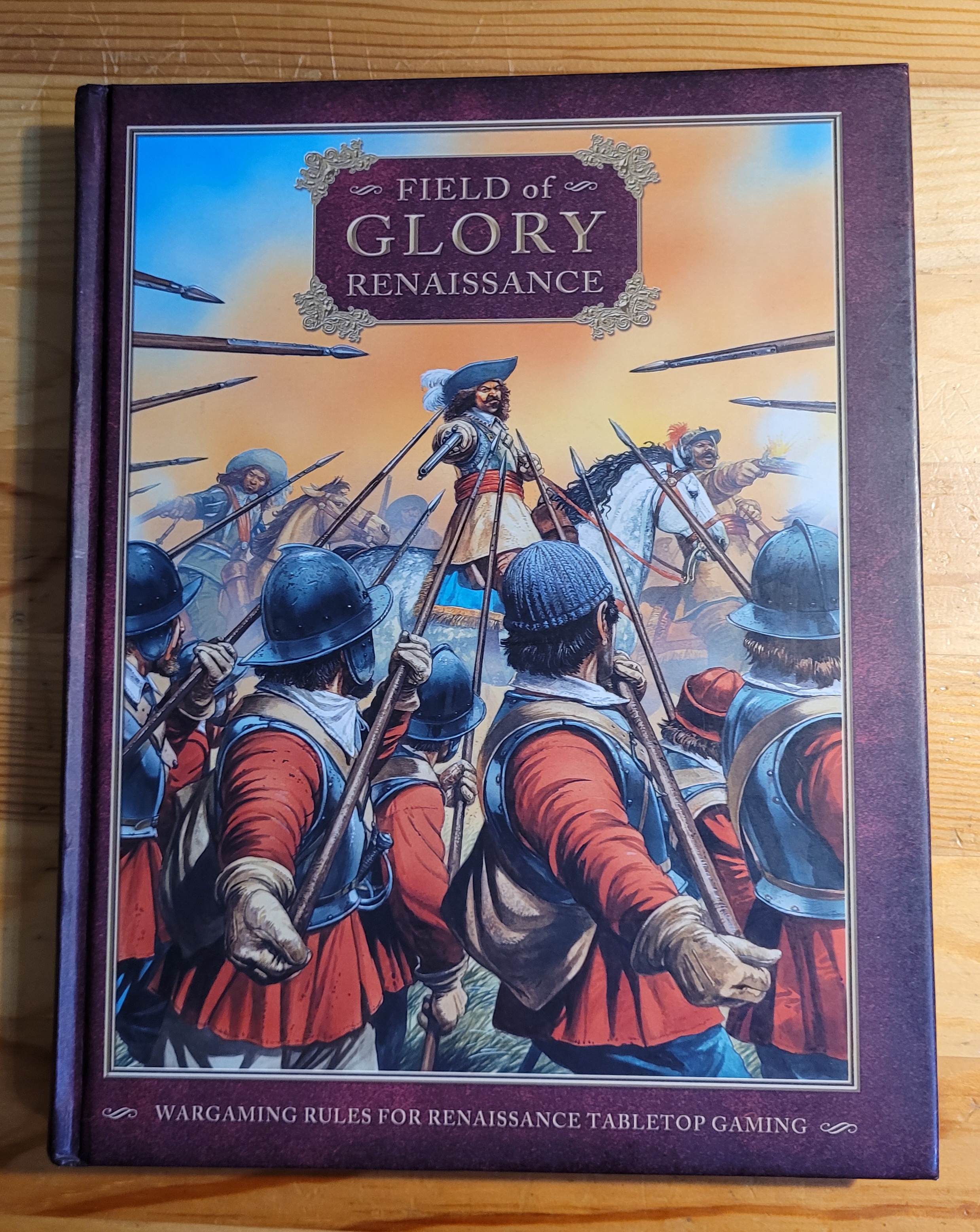The image depicts the front cover of a book titled "Field of Glory Renaissance," which focuses on wargaming rules for Renaissance tabletop gaming. The book, which has a brown outline and is resting on a light wooden surface, features an intricate illustration. In the center of this cover, a man on a white horse is prominently visible, pointing a gun at a group of soldiers surrounding him. These soldiers, reminiscent of Spanish conquistadores, are dressed in traditional Renaissance attire, with red and blue clothing and blue helmets, and they are all armed with spears. In the background, two additional men on horseback also appear to be brandishing their weapons towards the soldiers below. The book's dark plum color adds to the rich, historical feel of the scene depicted. The title is positioned at the top center, while the subtitle, "Wargaming Rules for Renaissance Tabletop Gaming," is located at the bottom.